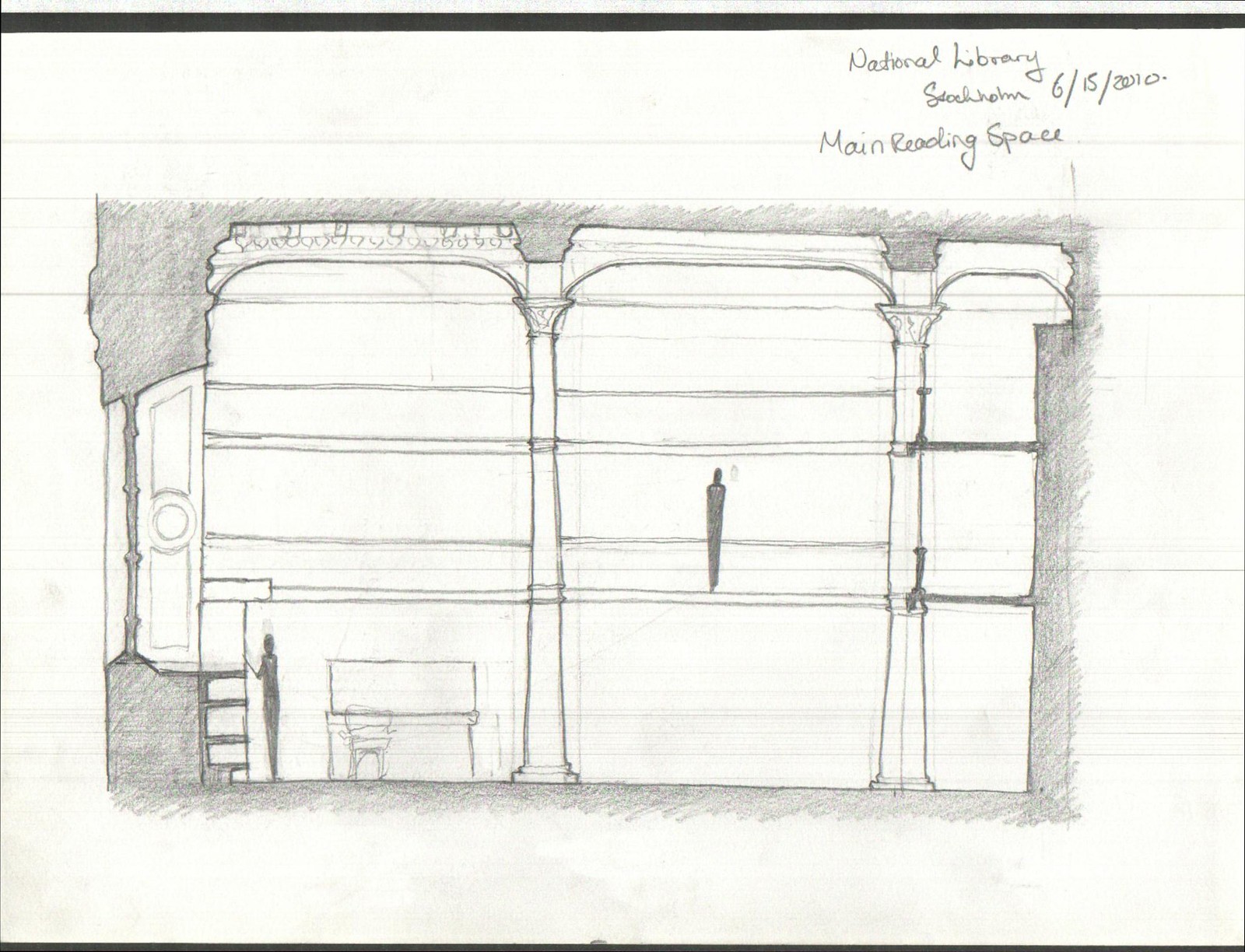This pencil illustration, titled "National Library, Stockholm" and dated 6-15-2010, depicts the main reading space of the library. The drawing features a gray background divided into four vertical segments, with the first segment being shorter than the others. Black handwritten text in the upper right corner identifies the location and date. 

In the illustration, the bottom floor shows a detailed scene: a person stands to the left with one arm resting against a wall with shelving. There's a desk with a chair nearby. The floor above, seen in the center segment, has a more abstract portrayal with a loosely sketched figure and no visible furniture. Decorative columns rise from top to bottom, adding architectural detail. Each vertical section is crossed by lines, creating a cohesive design throughout the piece.